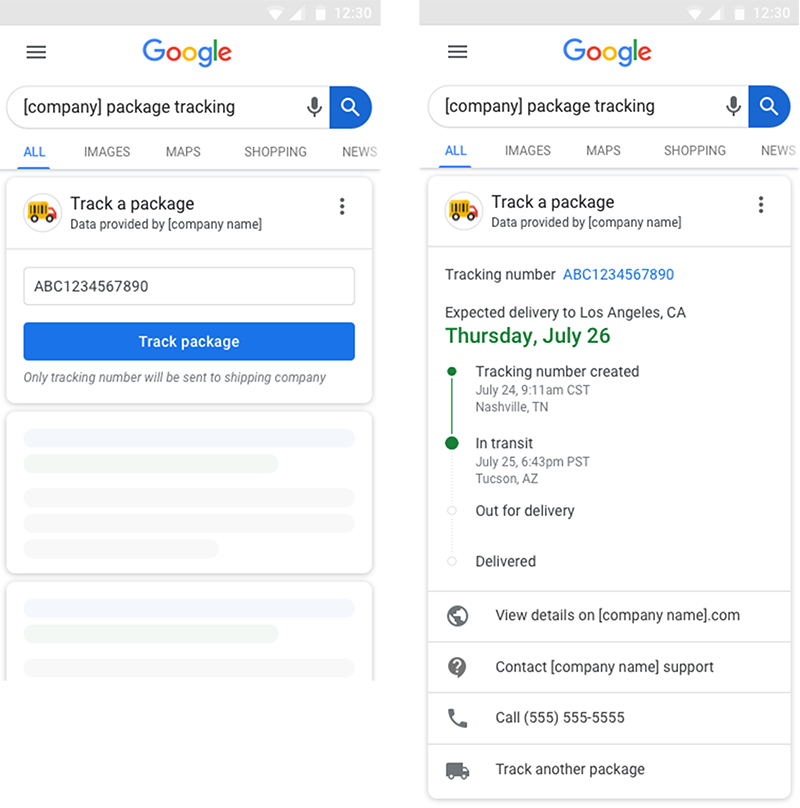The image is a side-by-side comparison of two screenshots showing a cell phone search related to package tracking on Google. The top part of both screenshots indicates they are Google searches. 

On the left-hand side, the search query is "Company Package Tracking." Beneath the search bar, options such as "All, Images, Maps, Shopping, and News" are visible. Below these options, a section for "Track a Package" appears, with a placeholder text field labeled "Data Provided for [J Company Name]." Within the text field, the tracking number "ABC1234567890" is entered, accompanied by a clickable button labeled "Track Package." A note clarifies that only the tracking number will be sent to the shipping company.

The right-hand side shows the results after the tracking number was entered and the search button was clicked. The top is consistent with the left side, displaying the three-bar menu icon and the word "Google." Below this, the interface updates to a "Track Package" section indicating the package's status. Specific details include an expected delivery location of Los Angeles, California, with an anticipated delivery date of Thursday, July 26th. Further down, the screen shows that the package is currently in transit and marked as "out for delivery."

This descriptive caption highlights a search query and subsequent tracking status for a package, demonstrating how users can locate and track shipments using Google on their cell phones.